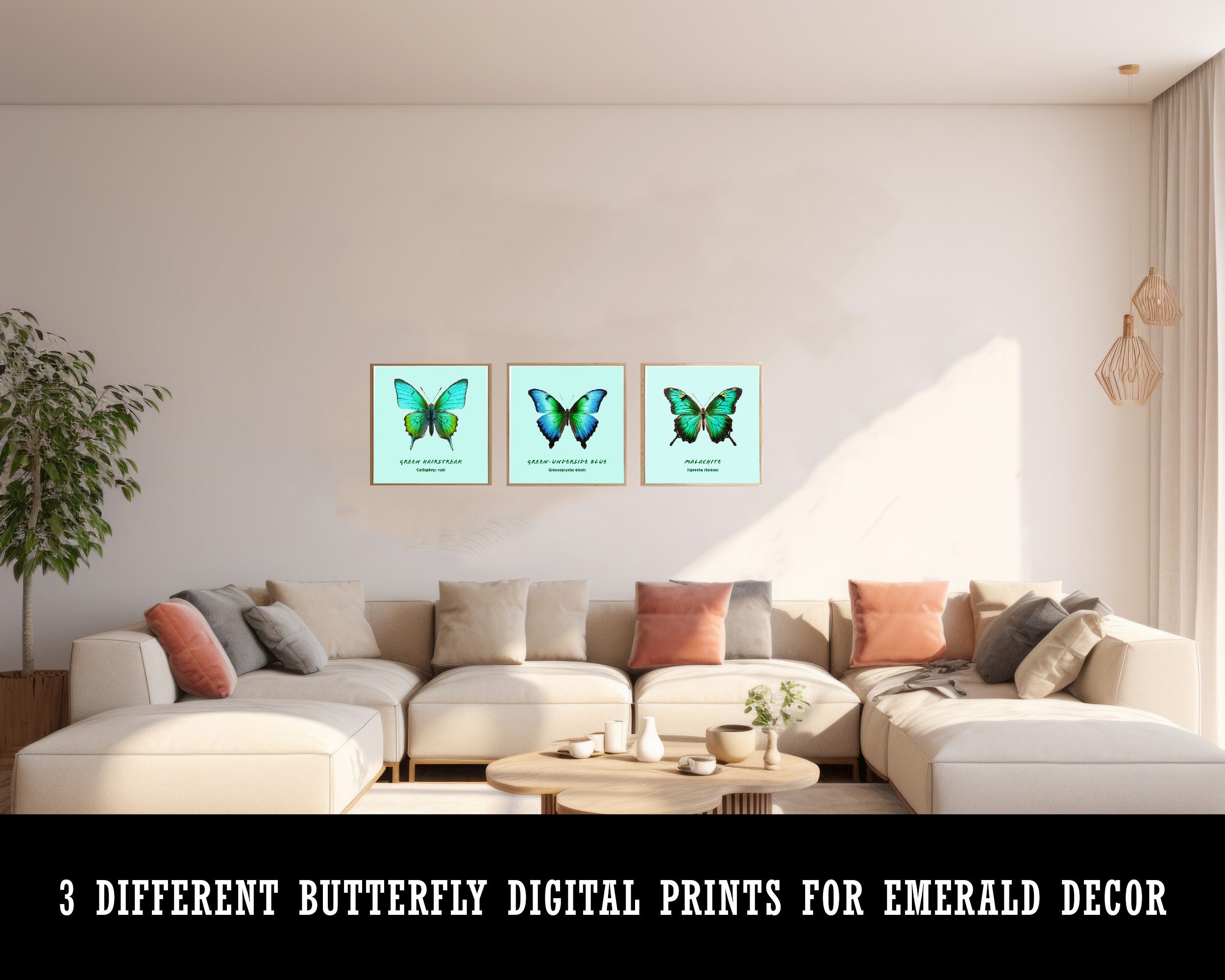This image showcases a beautifully decorated, beige-toned living room, highlighted by three distinct butterfly digital prints designed for Emerald Decor. These prints, which blend shades of blue, green, and black, are prominently displayed on a beige wall, enhancing the room's neutral color palette. The living room features a large cream-colored couch adorned with an assortment of pillows in tones of beige, tan, gray, and a hint of muted red and orange. There is also a coffee table, various seating options, and a potted plant to the left. Drapes adorn the right side of the room, adding to the overall cozy and elegant ambiance. A black banner with white text at the bottom of the image reads: "Three Different Butterfly Digital Prints for Emerald Decor."